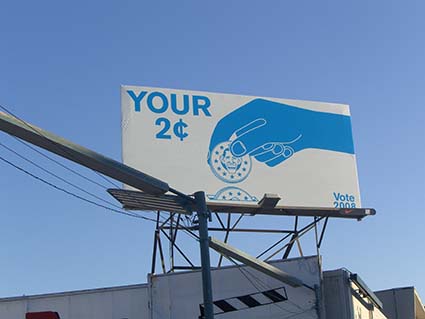In this outdoor image, a bright, cloudless blue sky stretches across the background, providing a serene, open atmosphere. The sunlight casts a radiant glow on the tops of two buildings, a small portion of which is visible. The buildings, standing at roughly the same height, form a noticeable corner. On one of the buildings, there is a distinctive rectangular sign with black and white stripes. Dominating the skyline is a massive billboard mounted on the rooftop of a building. The billboard features the message "Your Two Cents" in bold blue letters, accompanied by an illustration of a blue hand dropping pennies into a receptacle. Below the illustration, the text "Vote 2008" is prominently displayed, making it clear that this billboard was part of a campaign to motivate citizens to participate in the 2008 election by sharing their opinions through voting.